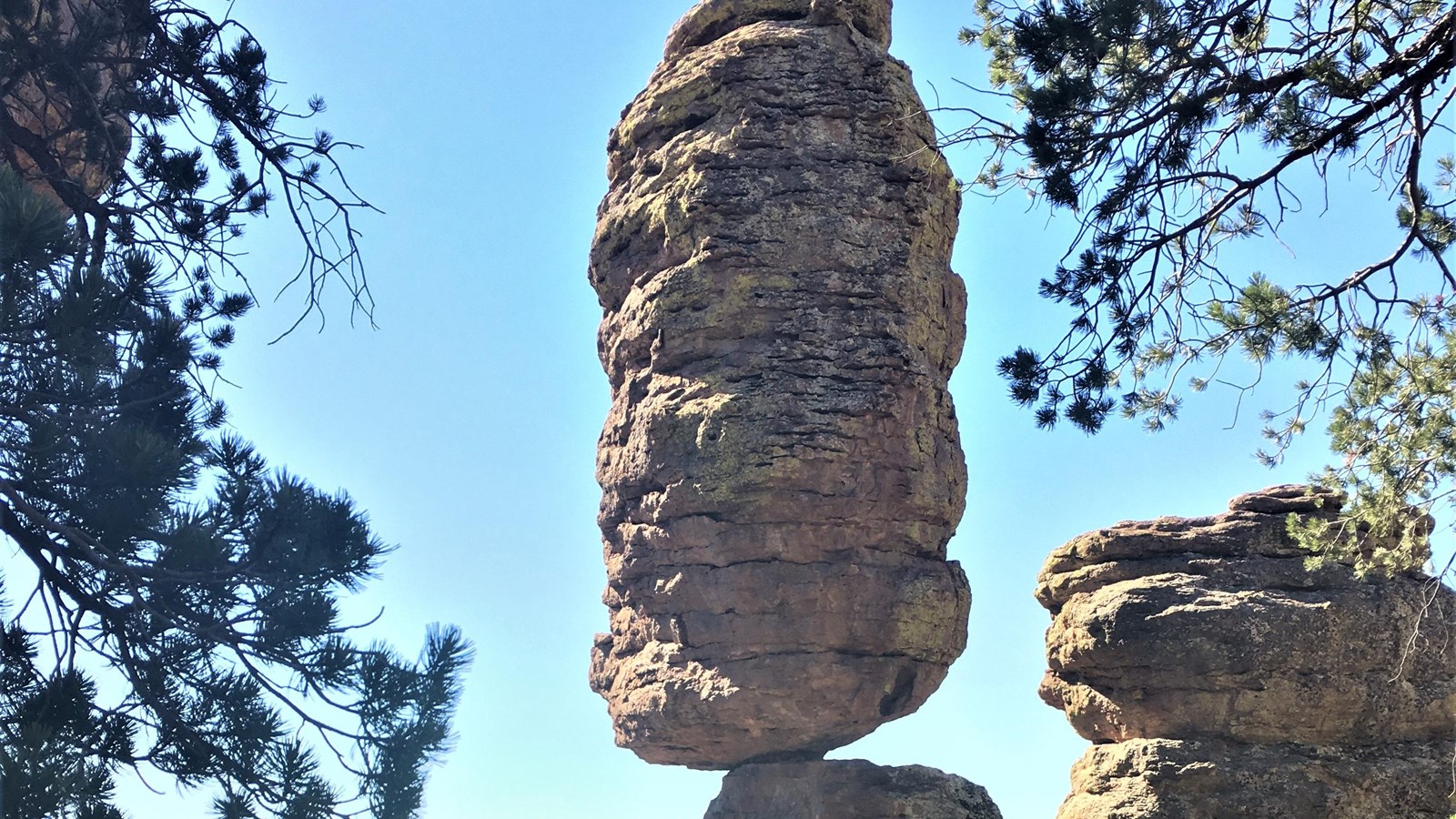This image showcases a striking natural rock formation, possibly taken in a National Nature Reserve. The scene presents a large, vertically oriented tan rock with numerous grooves, precariously balanced atop another smaller rock pedestal in the center of the photograph. The imposing rock appears as though it could topple over at any moment, yet it remains stable. On the right side of the image, more similarly colored rocks are visible, along with a tree adorned with abundant green leaves. To the left, there is another tree or bush with spiky leaves. The background features a clear blue sky with minimal cloud cover, enhancing the natural beauty of the scene. Sunlight illuminates the landscape from the left, casting a serene and vibrant atmosphere.